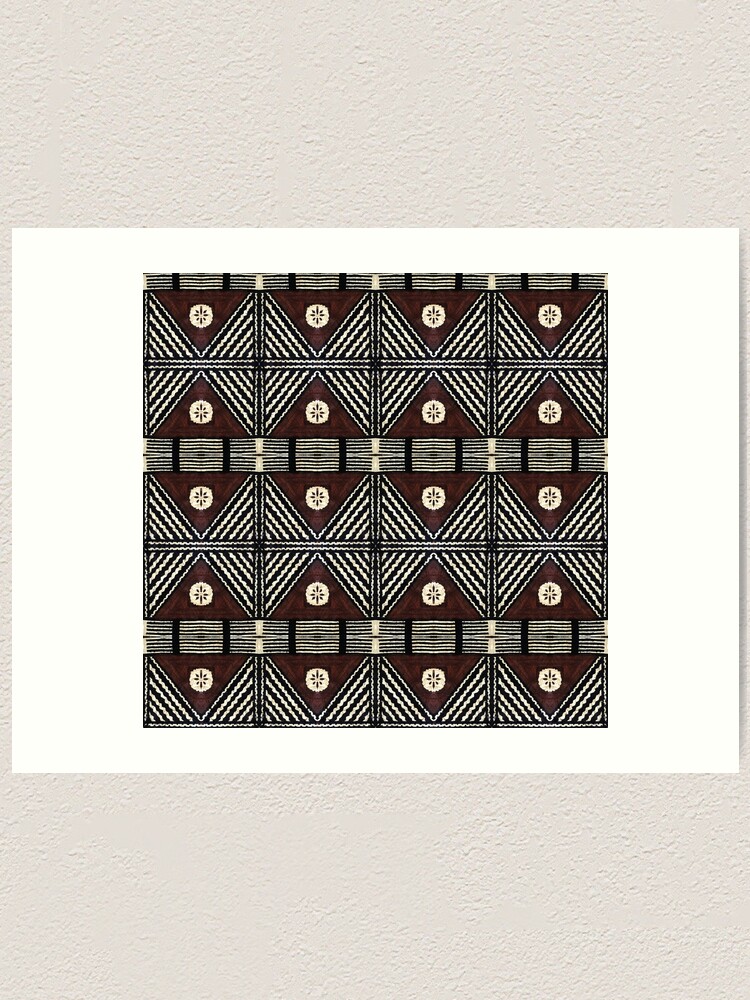The image is a highly detailed photograph showcasing a Fijian tapa cloth adorned with rich colors and intricate patterns. The cloth features a repeating design composed of black, beige, and maroon hues. The central pattern is arranged in a grid format with four columns and three rows. Each rectangular block maintains consistency in its intricate design: a maroon background with a white sand dollar at its center, intersected horizontally by black and beige lines. These lines are flanked by side-oriented triangles meeting in the middle, creating a harmonious visual effect. Notably, each row alternates, showcasing the triangles in an alternating orientation, which contributes to the illusion of interconnected diamonds. The overall image, appearing to be laid on a textured beige surface, emphasizes the fabric-like, textured nature of the tapa cloth, adding depth and a tactile quality to the visual experience.